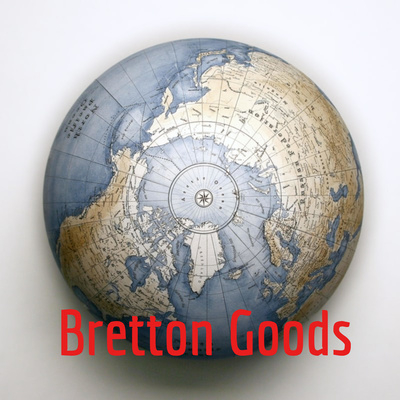The image features an advertisement for Breton Goods, prominently showcasing a globe as its central element. The globe, characterized by blue oceans and white or beige landmasses, is displayed from a top-down perspective, with the North Pole at the center. Superimposed in red text at the bottom of the image are the words "Breton Goods," emphasizing the brand name. The globe casts a shadow on the floor beneath, reinforcing the three-dimensional aspect of the representation. A small compass icon is also visible at the top of the globe. The background is predominantly white, drawing the viewer's attention entirely to the globe, hinting at a possible focus on selling this globe model at Breton Goods.